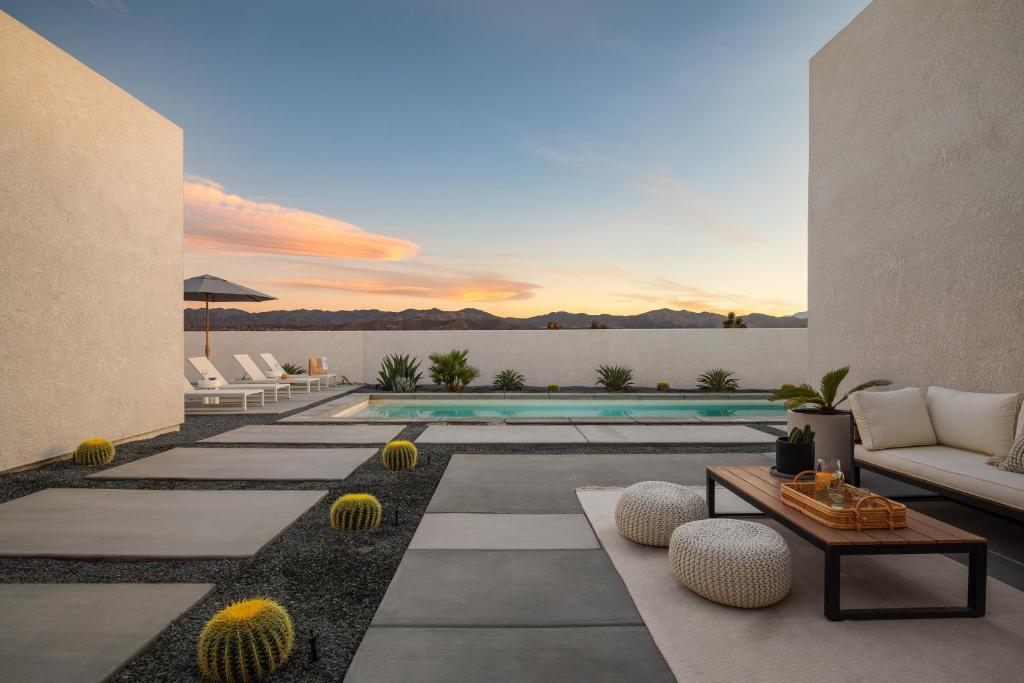The photograph captures a sophisticated outdoor space atop a building, potentially part of a luxurious home or a resort. The foreground features a stylish patio composed of large, square concrete slabs interspersed with contrasting black gravel. Centered on the patio is a sleek white couch with a black frame, complemented by a brown wooden coffee table also framed in black. The coffee table is adorned with two plants and a basket containing glasses. Flanking the table are two white cushion seats, providing additional seating.

To the right of the patio, the landscape transitions into a garden space with small, round cactuses embedded in the gravel. Two tall white walls rise on either side of the scene, creating a sense of seclusion and directing the viewer’s gaze toward the background.

In the backdrop, an inviting, perfectly rectangular pool stretches out, bordered by white lounge chairs and a solitary gray umbrella. The pool area exudes modernity and meticulous design. Beyond this lies a white wall that separates the immediate outdoor space from a distant view of mountains, which stand majestically under a sky painted with pinkish-orange clouds, suggesting a picturesque sunset. This harmonious blend of architecture, nature, and sky suggests both tranquility and sophistication.